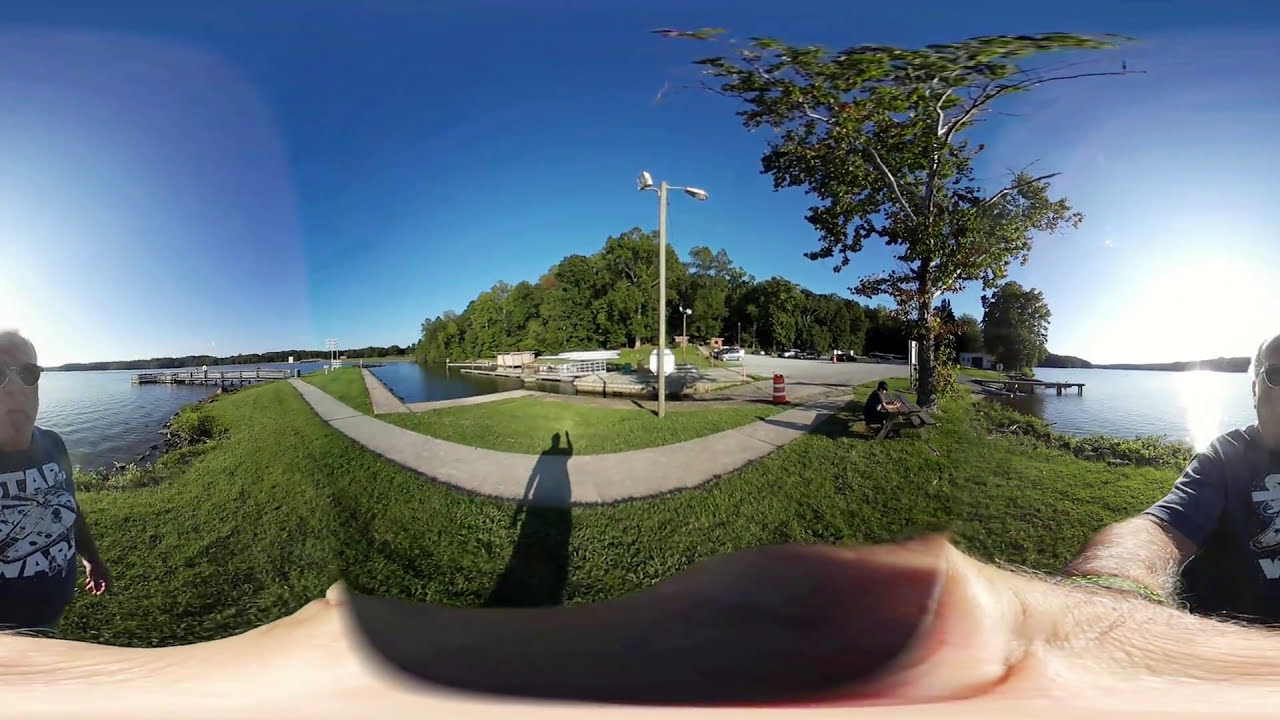In this panoramic outdoor photograph taken during daytime, the lush greenery of a natural park area is prominently featured alongside a bluish water body. A wooden pier extends into the lake from the left side, while trees with vibrant green leaves frame the scene. A central sidewalk, curving in the image due to panoramic distortion but likely straight in reality, leads towards the pier. A light post with a traffic cone nearby stands in the center, acting as a subtle focal point. The clear blue sky suggests the sunlight is strongest on the right side of the photo. A person seated at a picnic table on the right adds to the tranquility of the setting. In the foreground, a man wearing sunglasses and a Star Wars shirt is taking a selfie with a camera held out in front. His image is mirrored on both the left and right sides of the panoramic image, emphasizing the unique wrap-around effect of the photograph. The scene in the background aligns seamlessly with his position, creating a harmonious blend of nature and human presence.